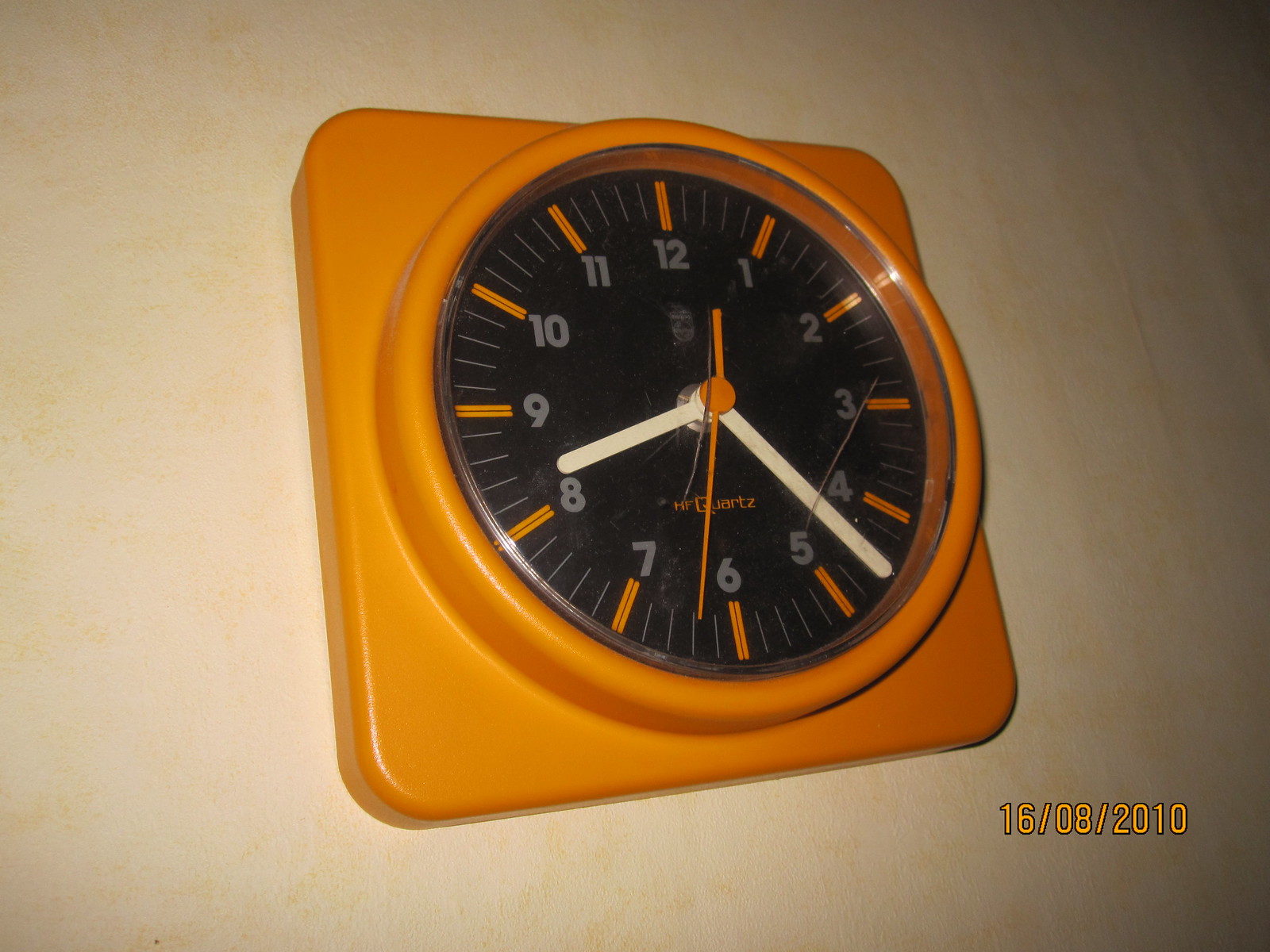This vintage wall clock, possibly from the 1950s or 1960s, features a distinctive mid-century design. The clock's square silhouette has smoothly rounded edges, with a base platform approximately half an inch thick. Its background, crafted from an orangey-tan plastic, seamlessly blends nostalgia and simplicity. Set into the center of this background is a circular frame in the same tan hue, housing the actual clock face. The face itself is characterized by black with white hands and orange ticks marking the hours and minutes. The detailed ticks and numbers ensure precise timekeeping, making this clock both a functional timepiece and a charming retro decor piece.